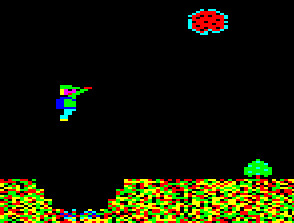In this highly pixelated screenshot from an old-school video game, a character is captured in mid-air, seemingly jumping over a large, oval-shaped gap in the ground. The ground itself is composed of various multi-colored blocks, including shades of yellow, green, red, and black, forming a jagged, edgy landscape. The character, depicted with a square head and blocky features, wears a blue suit, a dark blue backpack, a green hat, and has yellow hair. They are holding something red in their hand, possibly a gun. The background of the image is entirely black, emphasizing the contrast. In the top right corner, there appears to be a round object with white or blue edges, red in the center, and black dots. A small green tree sits at the bottom right, adding a touch of nature to the otherwise stark scene.